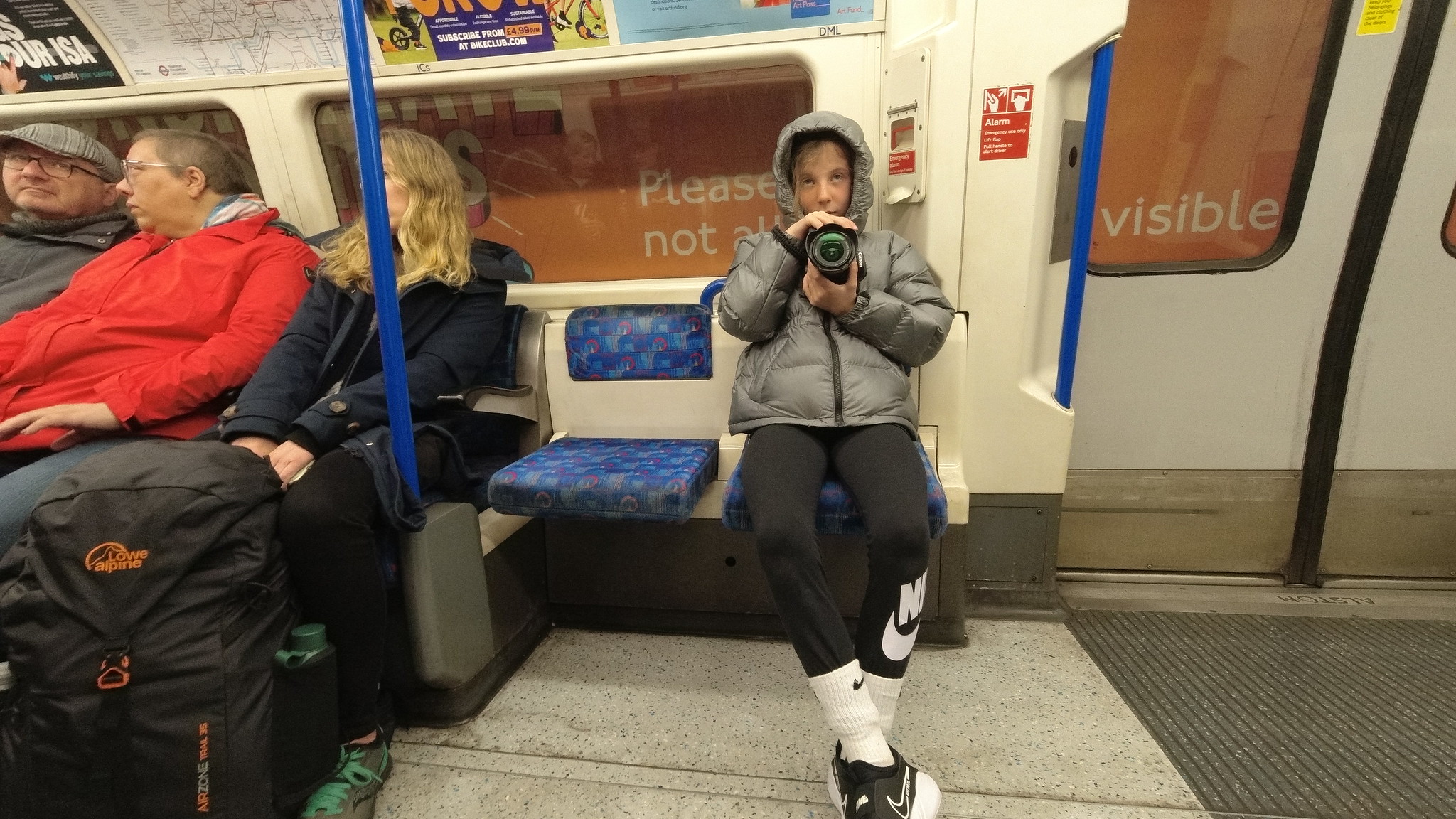The image captures the interiors of a subway car teeming with different colors and textures. Dominating the center of the photo is a young girl sitting on a blue seat to the right, draped in a gray puffy coat with the hood up. She sports black Nike pants, white Nike socks pulled up to her calves, and black and white Nike shoes. The girl holds a black camera aimed directly at the photographer, whilst she gazes slightly upwards. Adjacent to her, on her left, is an empty blue seat, and further left, there are three other passengers seated, dressed in a variety of coats in colors like black, gray, red, and blue. One woman has a black and orange backpack with a green water bottle. The floor of the car features a carpet-like material near the doors. In the background, subway advertisements, one mentioning "subscribe for $4.99 at bikeclub.com," decorate the area above the windows. The setting vividly showcases an ordinary moment of subway life, punctuated by the vibrant attire of the passengers and the eclectic shades of the seats and environment.